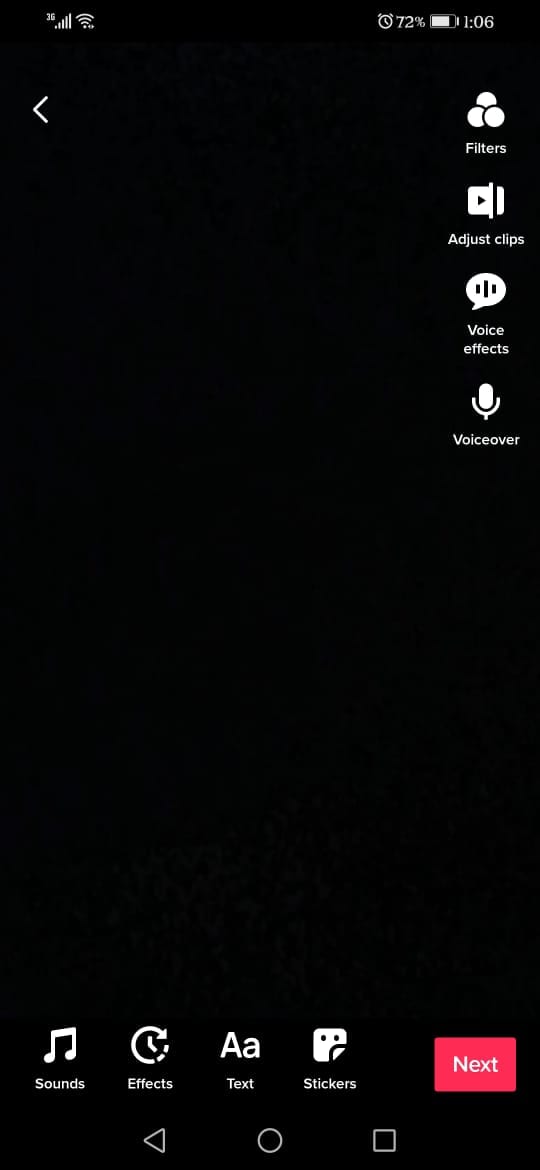A cell phone screenshot is displayed against a solid black background. The upper right corner of the screen shows an alarm clock icon, a battery indicator at 72%, and the time 1:06. In the upper left corner, there are five signal bars indicating full reception, a '3G' label, and a Wi-Fi icon indicating connectivity.

On the right side of the screenshot, white text with corresponding icons display options such as Filters, Adjust Clips, Voice Effects, and Voiceover, arranged vertically. At the bottom of the screen, from left to right, there are icons and labels for various functions in white text: 'Sounds' with a musical note icon above it, 'Effects,' 'Text' with a capital and lowercase 'A' icon, and 'Stickers' with a square face containing two eyes. Towards the far right, there is a red action button labeled 'Next.' Below all the options, the home button is centered at the bottom of the screen.